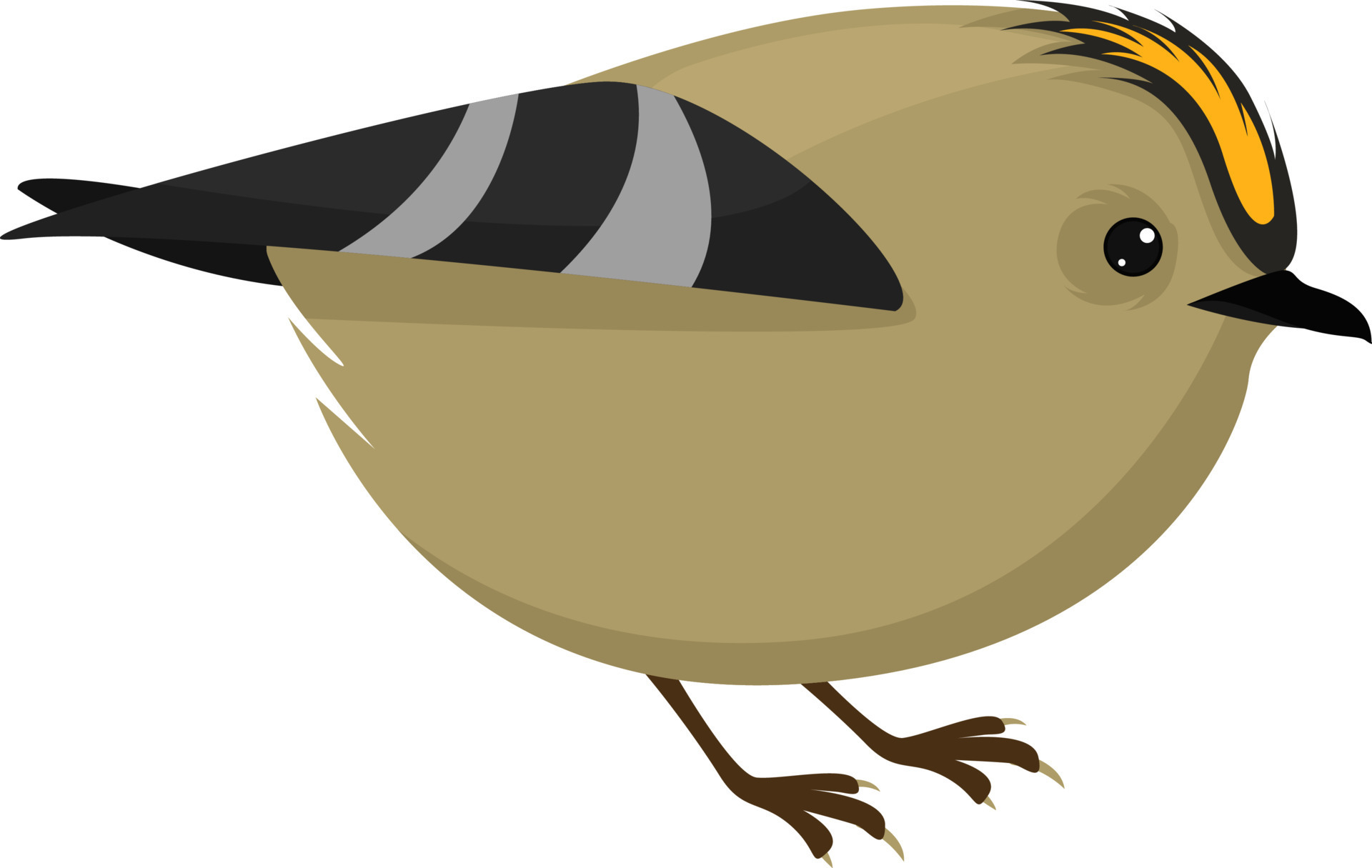The image depicts a simplified, clipart-style illustration of a plump, medium brown bird standing upright against a white background. The bird is shown in a side view, facing to the right with its tail to the left. Its head features a short, black beak and a black eye with a white reflection. A distinctive yellow crest, bordered in black, extends from between the bird's eyes up to the top of its head. The wings, colored black and folding back past its tail, display two prominent gray stripes. The bird has dark brown legs, each foot with three toes that are adorned with light brown claws. The edges of the bird's body are slightly darker brown, contributing to a flat, minimalistic aesthetic with some subtle shading.